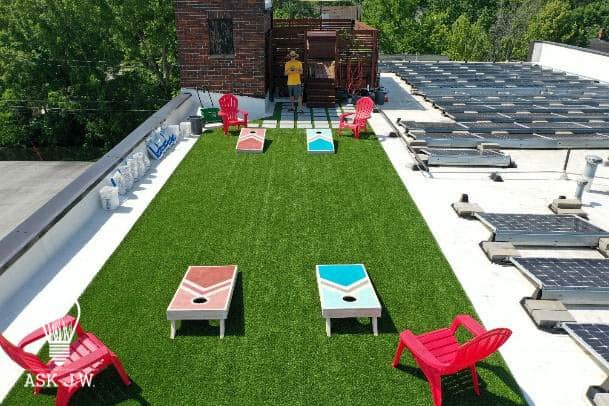The image captures a detailed rooftop scene. The roof is painted white and features a large rectangular area covered in green artificial turf. Situated at each corner of this turf are four red plastic lawn chairs. Both ends of the turf area host sets of cornhole boards—one pair colored red and light pink and the other blue and light blue—arranged for gameplay. A man in a yellow t-shirt, green shorts, and a sun hat stands in front of the cornhole games.

To the left of the turf area, there's a small room with brick walls adjacent to a wooden deck, which likely serves as an entry point to the roof. On the right side of the roof, a substantial section is filled with around 100 solar panels. Along the perimeter, near the banister, there are bags and buckets containing various items. In the background, outside the rooftop area, a grove of trees and power lines can be seen.